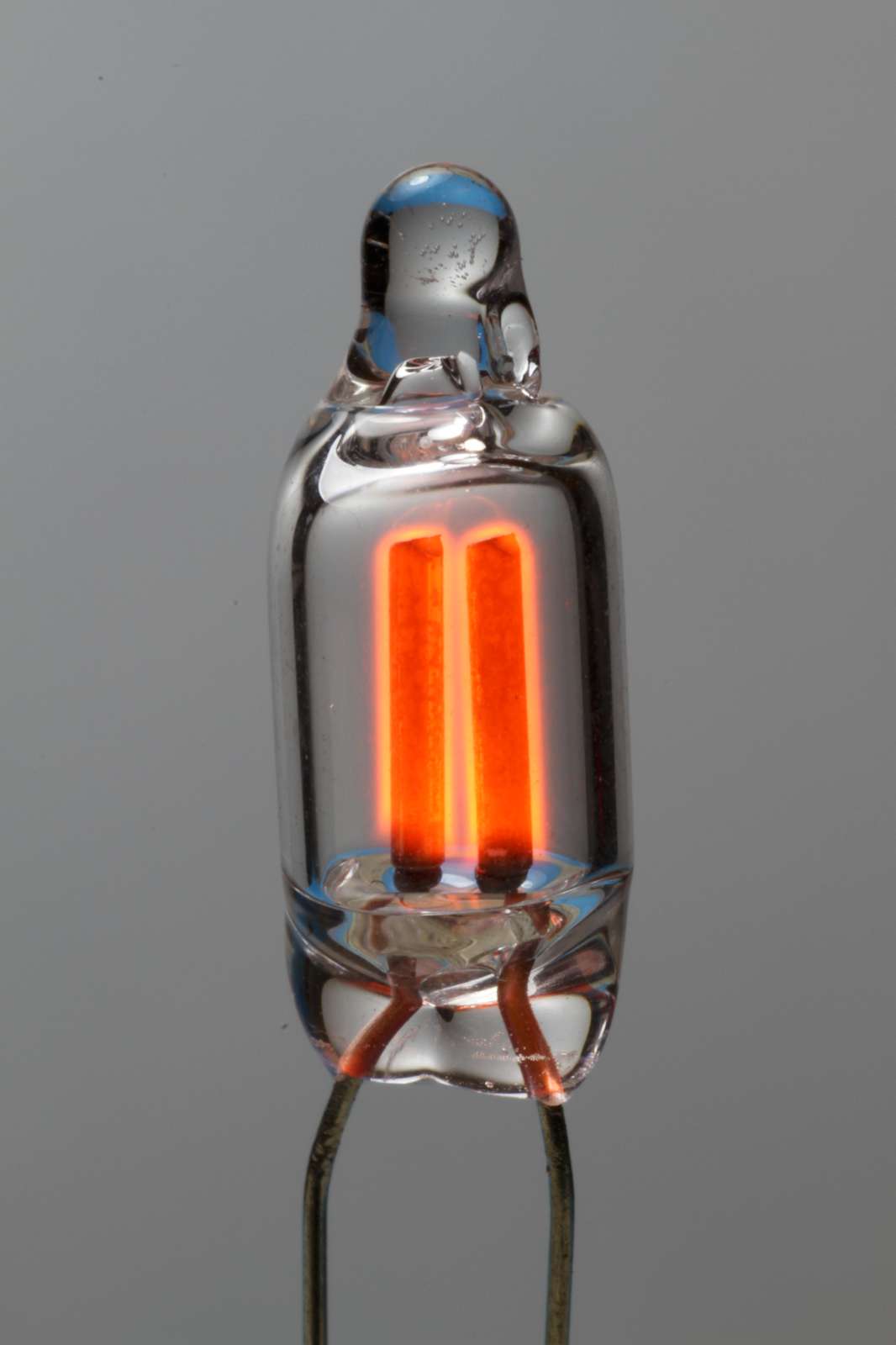The image depicts a close-up view of an unusual and intriguing object resembling a heating element or fuse within a rectangular glass container. The background is a medium gray, providing a stark contrast that highlights the details of the object. The container is an oval metal structure, reflecting its surroundings and displaying some condensation at the top, making it appear slightly wet. Inside the glass, centrally located, are two vibrant, fiery-orange and yellow elements that resemble hot, glowing antennas, suggesting a high temperature. These elements appear to radiate heat or electricity, contributing to their intense coloration and seeming motion. Extending from the bottom of the unit are wires, transitioning from bright red copper at the top to green and black towards the base, where they connect to the heating elements. The intricate and reflective design of the structure, with its combination of metal and glass, gives it a distinctive and somewhat artistic appearance.